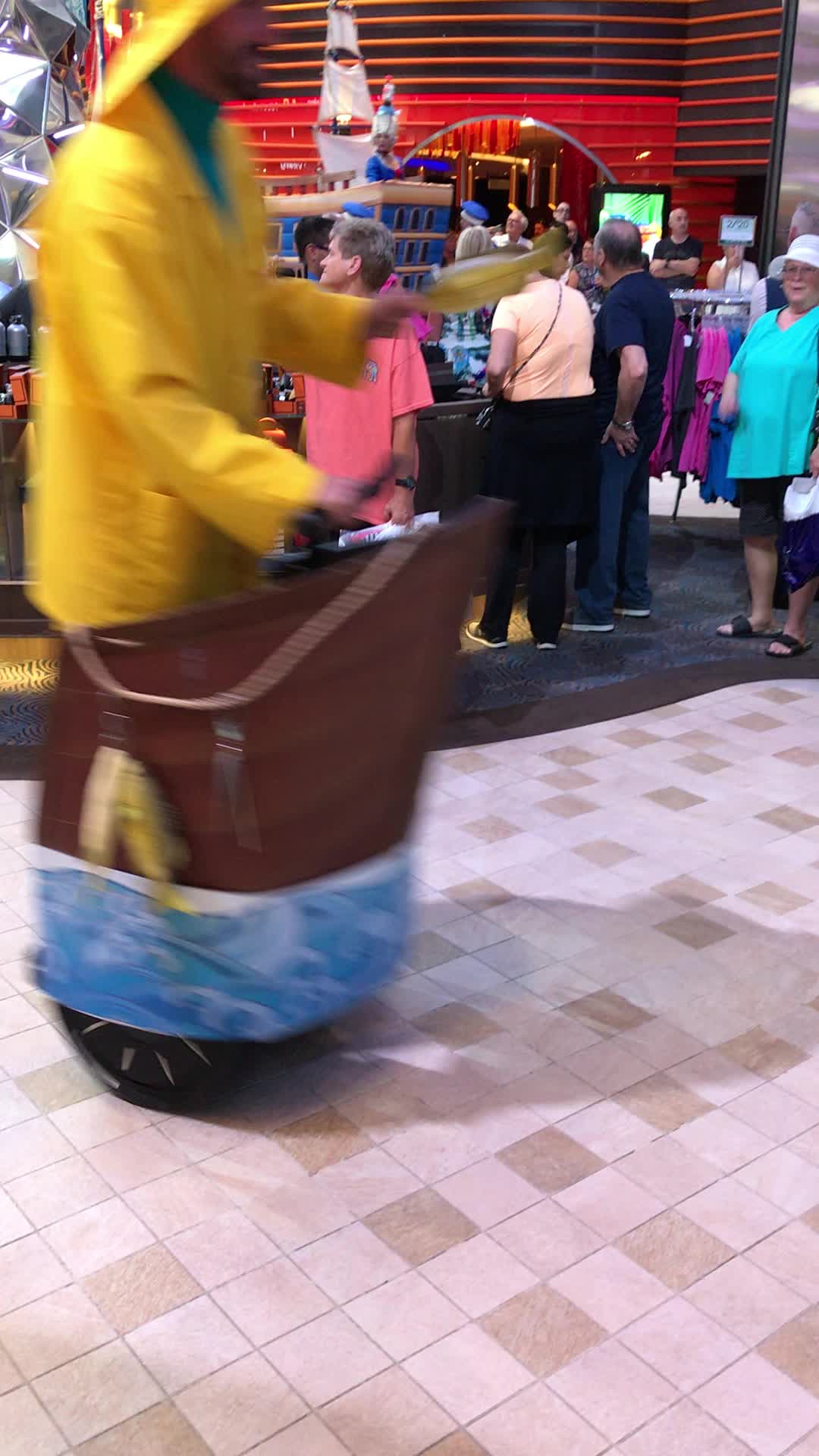The image captures a lively scene set in what appears to be a gift shop or resort store, centered around a quirky and somewhat humorous figure. In the foreground stands a man dressed in a yellow raincoat and matching yellow hat, reminiscent of the fisherman on a fish stick box. He is blurry in the photo but unmistakably prominent. The man appears to be riding a decorated Segway designed to look like the front of a boat, complete with a fishing line and fish, and the bottom painted to resemble water. This setup amusingly contrasts with the setting.

Beside him on the floor is a small statue or figure with a black base, a blue middle, and a dark brown top. Toward the right, a woman in a turquoise shirt, black culottes, and black sandals, capped with a white hat, looks towards the man in the raincoat. Behind her, another woman in a yellow shirt and black pants stands next to a man in black shirt and pants, seemingly engrossed in something.

The background reveals a vibrant red and black striped wall and a couple of racks laden with pink and blue t-shirts. Some people are casually perusing the merchandise while others stand around, adding to the busy and out-and-about atmosphere. Way in the background, there's a hint of a larger decorative element resembling a pirate ship. Overall, the image exudes a bustling, almost whimsical feel with people dressed both in costumes and regular attire, blending into the lively environment.